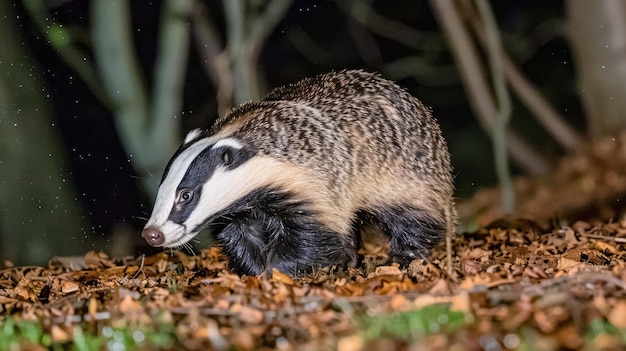This detailed photograph captures a cute badger shuffling through a forest floor covered in orange-brown dead foliage, with a few patches of green grass and leaves visible. The badger has a distinctive black-and-white striped face, reminiscent of both a skunk and a weasel, with a chocolate brown snout and whiskers. Its coat features a unique mix of light brown and black fur, with its lower body and legs cloaked in jet black, giving it a quirky yet endearing appearance. The badger, seemingly unaware of being photographed, is looking off into the distance towards the bottom left corner of the image. The background is softly out of focus, highlighting branches and trees, which adds depth to the scene and reinforces the natural woodland setting. The badger's stance and the surrounding elements suggest it might be a nocturnal creature caught in a candid moment.